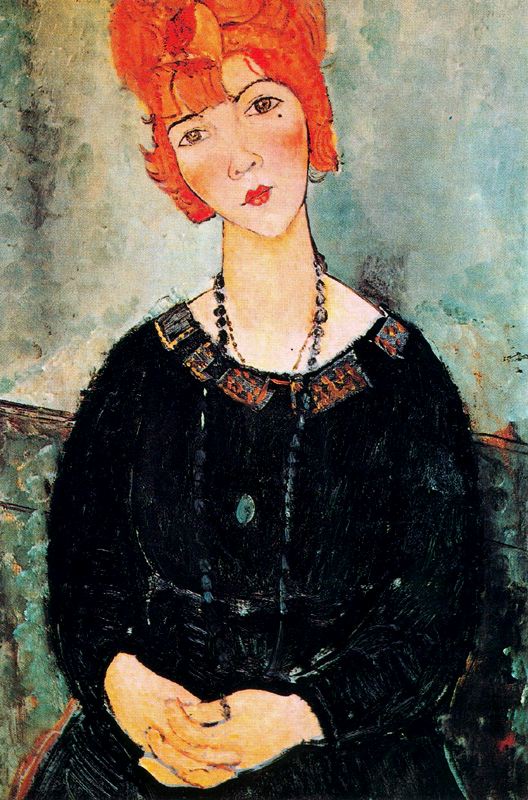The image is of a painting portraying a fair-complexioned woman with bright red hair styled elaborately upwards. She has striking green eyes, a small red mouth, and is adorned with makeup, including prominent red lips and a mole beneath her left eye. The woman is attired in a black dress featuring blue buttons and intricate yellow and orange embroidery around the collar. She wears a long, dark beaded necklace that reaches down to her belly button, layered with a smaller gold necklace. Her hands, which are clasped together on her lap, display a thumb ring on her right thumb.

The background behind the woman is a stylized mix of colors, with the upper section featuring blue, tan, and gray hues, and the lower portion, from her shoulders down, displaying shades of green, gold, and gray. The wall has an old, slightly stained texture that further adds to the painting's vintage feel. She is posing with her head slightly tilted to her right, conveying a poised and composed demeanor. The overall style of the painting is notably aged, giving the impression of a piece from a bygone era.